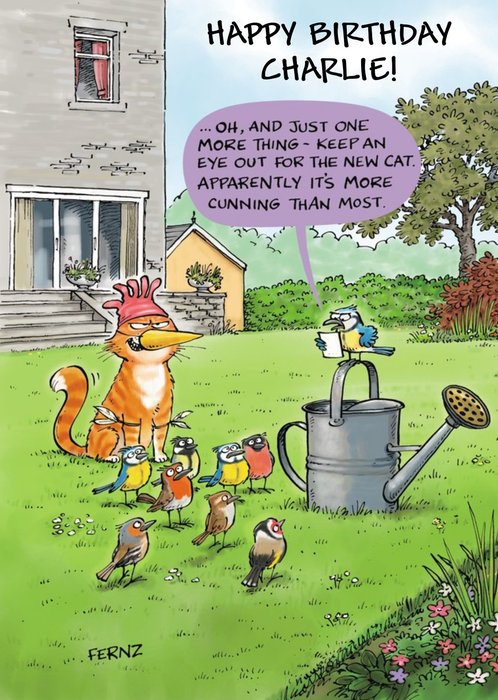This cartoon-style drawing, portraying a homemade birthday card, is set in a lush, green backyard with a blue sky, trees, and a variety of colorful birds. At the top right, in bold black text, it reads "Happy Birthday Charlie." In the upper left corner, a gray house with sliding doors, large windows, and a small cream shed is depicted. Below, on the lawn, a scene unfolds with a yellow cat disguised as a bird. The cat wears a bird’s beak, a red glove-like hat, and feathers tied around its front legs, giving it a cunning and mischievous appearance.

Surrounding the cat are birds of various colors – blue, yellow, red, and brown – intently listening to a small blue and yellow bird perched on a tin watering can. This bird is reading from a piece of paper and has a thought bubble saying, "Oh, and just one more thing. Keep an eye out for the new cat. Apparently, it's more cunning than most," adding a humorous twist to the scene. The overall illustration captures a playful and imaginative birthday greeting, drawing on the comedic elements of cartoon and comic strip art.